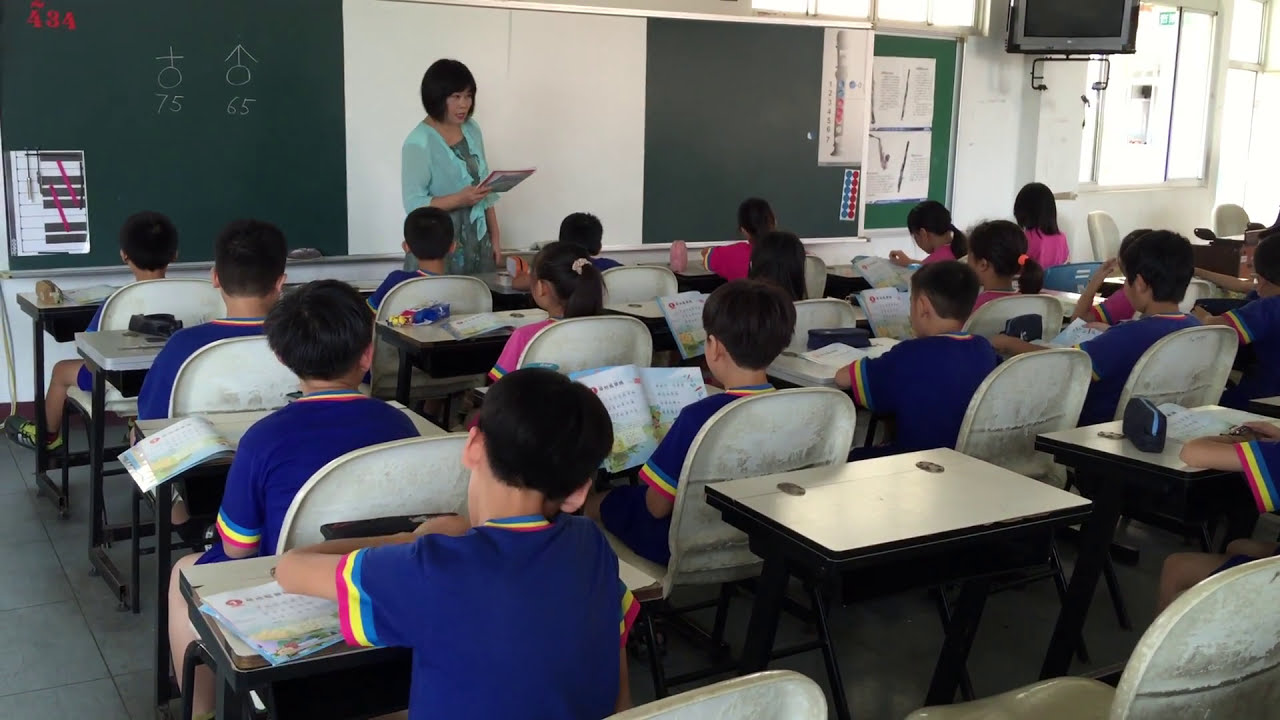In this detailed photograph of an indoor, daytime classroom setting, numerous students are seated at desks with white tops and corresponding white chairs. All the students are facing away from the viewer, engaged in study. The boys are uniformly dressed in blue t-shirts adorned with light blue, yellow, and red accents around the sleeves and collar. The girls, most sporting ponytails except for two with their hair slightly down, wear pink shirts featuring the same colorful trim.

At the front of the classroom, slightly to the center-left of the image, stands the teacher. She is attired in a turquoise blue shirt and a green dress, facing the class and indirectly the viewer. Behind her, there is a white drop-down board centrally positioned, flanked by green chalkboards on both the left and right. The left green board displays a white sheet of paper with red tags and black bars. To the right, another green board shows various instruments; the upper part features different kinds of oboes or clarinets, and the lower part displays a saxophone and a bass saxophone.

Additionally, there are some written details on the green chalkboards, including the number "75" under a female symbol, "65" under a male symbol, and "43a" in the upper left corner. A small accordion instrument and a red and blue sticker can also be seen on the right green board. The classroom is illuminated by natural light, suggested by the presence of a window in the top right corner of the image.